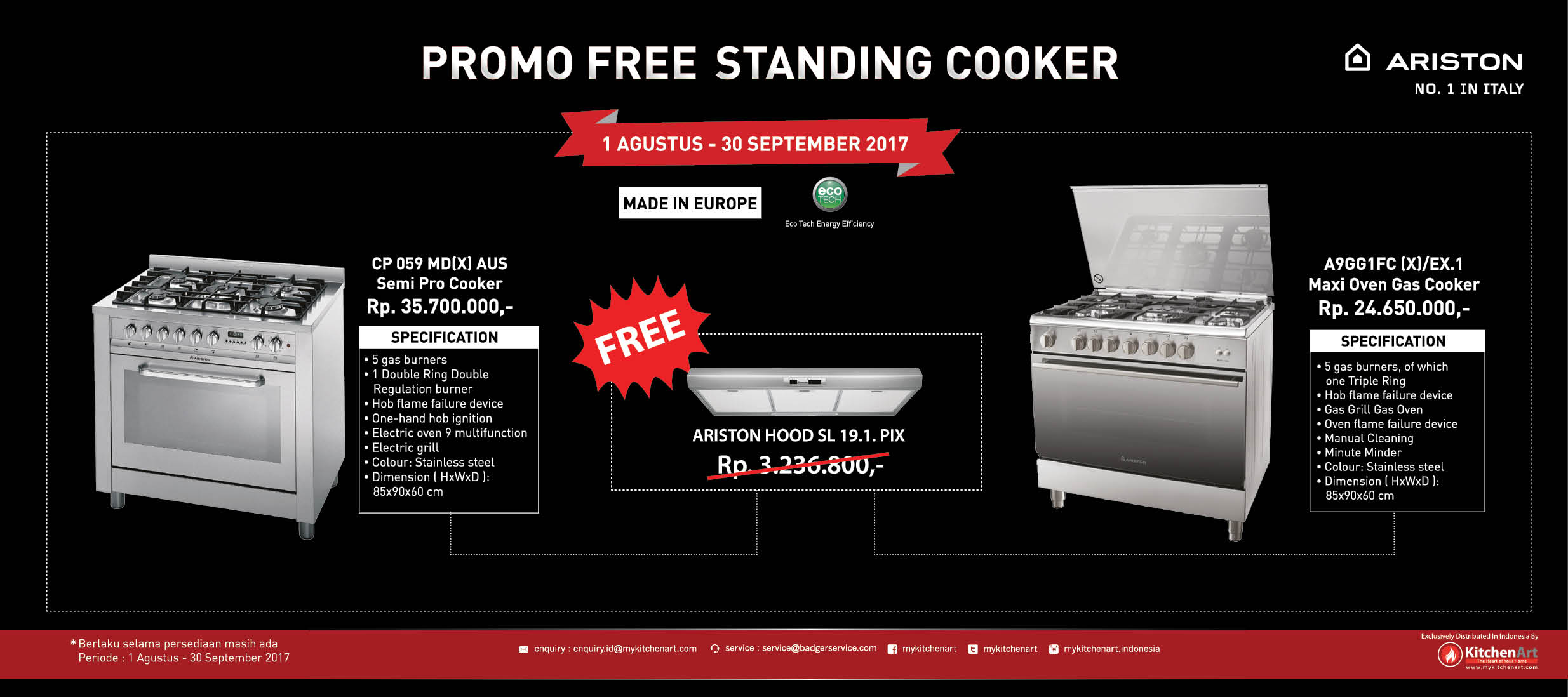The advertisement features a sleek black background accented with a maroon border at the bottom, containing some white text. At the top, bold white letters announce "Promo Freestanding Cooker." The ad prominently displays two cooking appliances: on the left is a semi-pro freestanding cooker with six burners and an oven complete with numerous knobs for various controls. On the right, another similar cooker is shown. Between these two cookers, there's an offer text in a red banner that reads, "Free Ariston Hood." The ad specifies that this promotion runs from 1st August to 30th September 2017 and highlights that the products are made in Europe. Additional details about specs and a complimentary hood are indicated, emphasizing the high functionality and quality of the Maxi Oven Gas Cooker from Airsten.